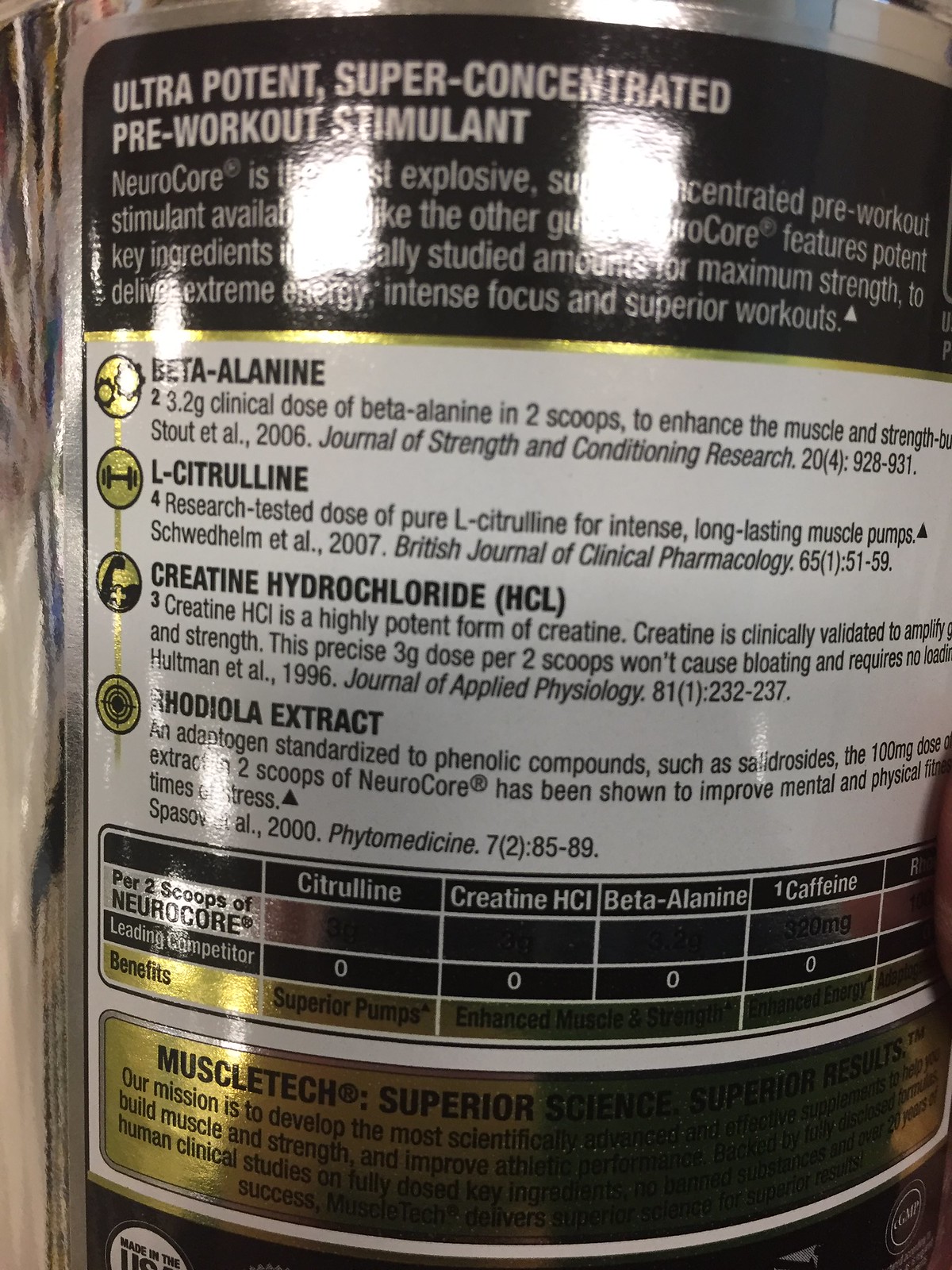This is the back label of a bottle containing a pre-workout stimulant called "NeuroCore." The top section of the label is black with bold, white text that reads "Ultra Potent Super Concentrated Pre-Workout Stimulant." Beneath this, the label transitions to a white background bordered by a gold band. Here, the list of ingredients is displayed in black lettering: beta alanine, L-citrulline, creatine hydrochloride, and rhodiola extract. Each ingredient is accompanied by detailed sentences describing its dosage and purpose. Further down, another black section features a graph, likely illustrating some aspect of the product’s efficacy or ingredient breakdown.